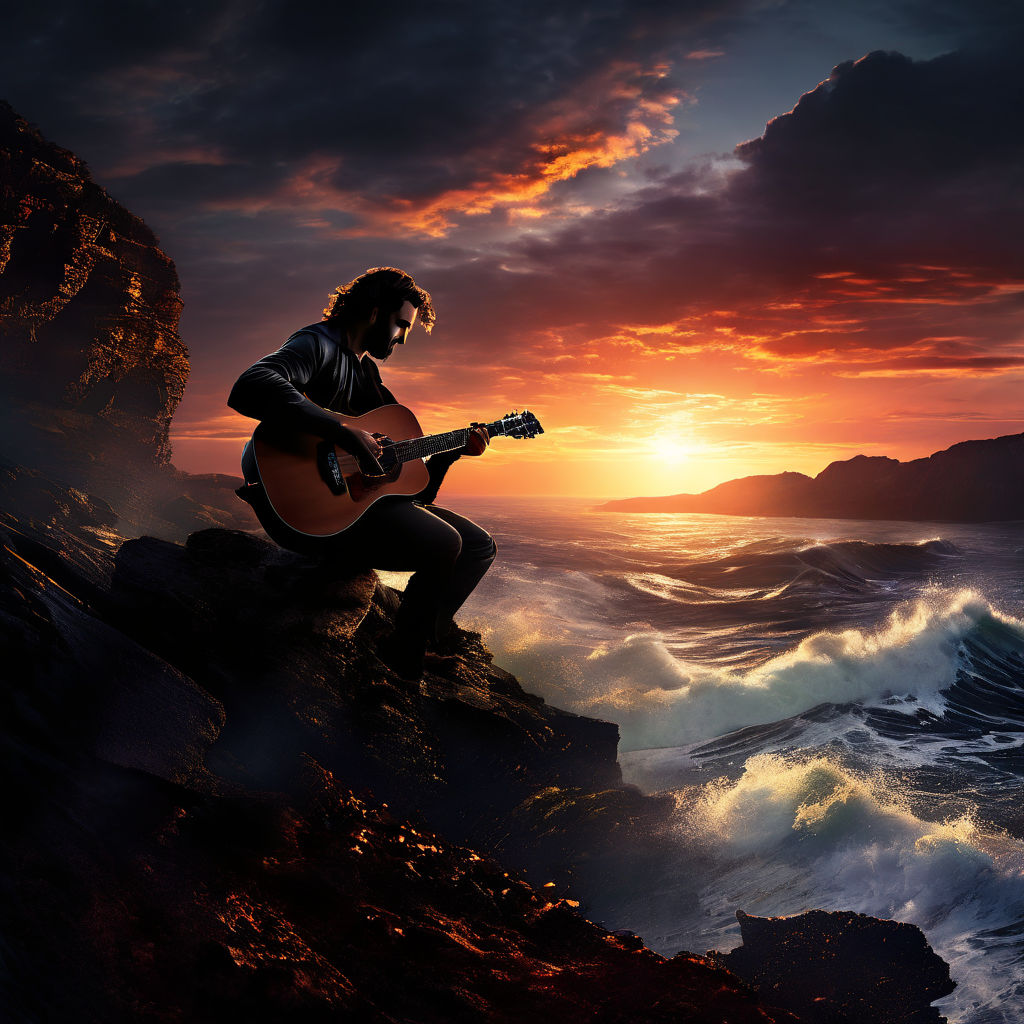The image portrays a serene coastal scene at sunset, where a man sits slightly left of center on a reddish-hued rocky shore, playing a brown guitar. His body is turned sideways, revealing only half of his figure. The setting sun, positioned in the middle right of the image, bathes the surroundings in warm shades of yellow, orange, and red. To the left behind the man stands a rugged cliff, while waves crash onto the rocks below in the bottom right corner. Dark clouds loom in the upper corners of the sky, adding contrast to the vibrant sunset colors and completing this tranquil, picturesque moment by the ocean.